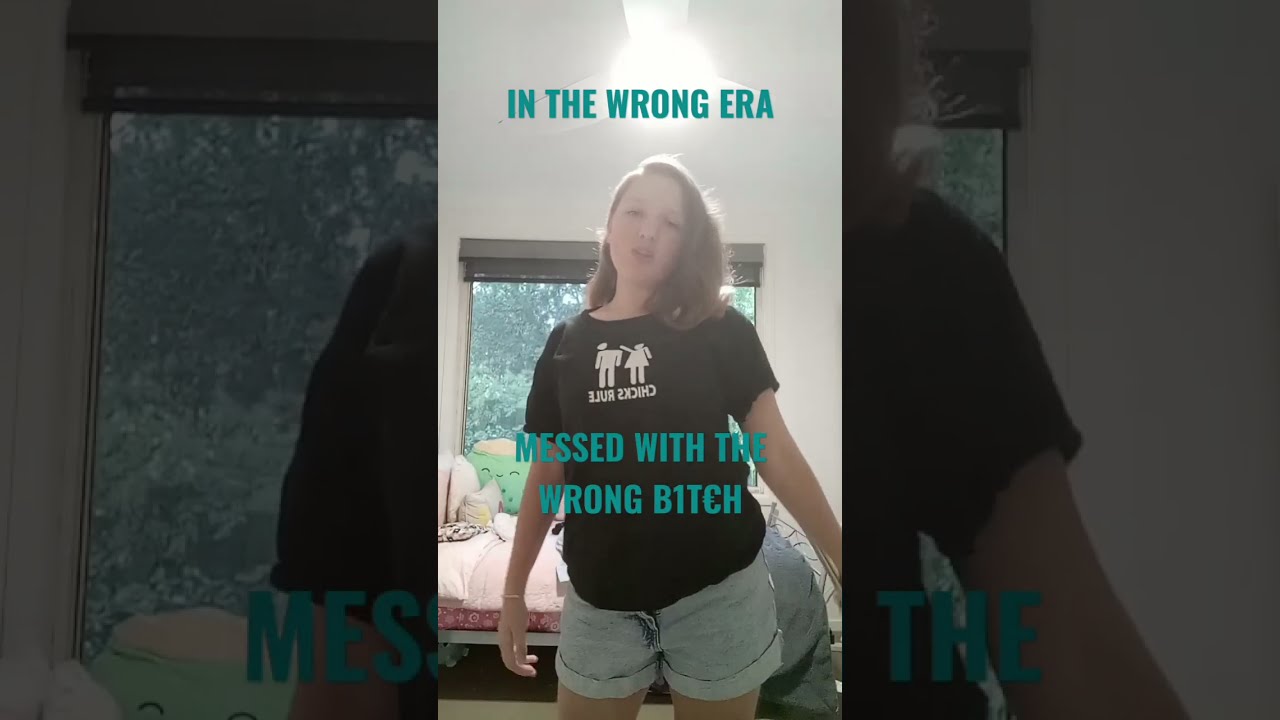The image depicts a Caucasian girl in her mid to late teens with shoulder-length light brown hair parted to the side. She appears to be somewhat overweight and is dressed in an oversized black t-shirt, which features white outline figures resembling bathroom signs. The female figure on her shirt is shown punching the head off the male figure, accompanied by the text "Chicks Rule". The girl is standing in her bedroom, on a gray carpet with a gray blanket-covered bed behind her. A window with a view of green trees and a yard can be seen in the background. The lighting in the room casts a highlight on her hair, while her face remains somewhat in shadow. Above her head, overlaying the image, the text "IN THE WRONG ERA" is displayed, and below her, the text reads "MESSED WITH THE WRONG BITCH". To the left and right of the central image are magnified and darkened insets, focusing on parts of her arms and the window, showing fragmented parts of the text.